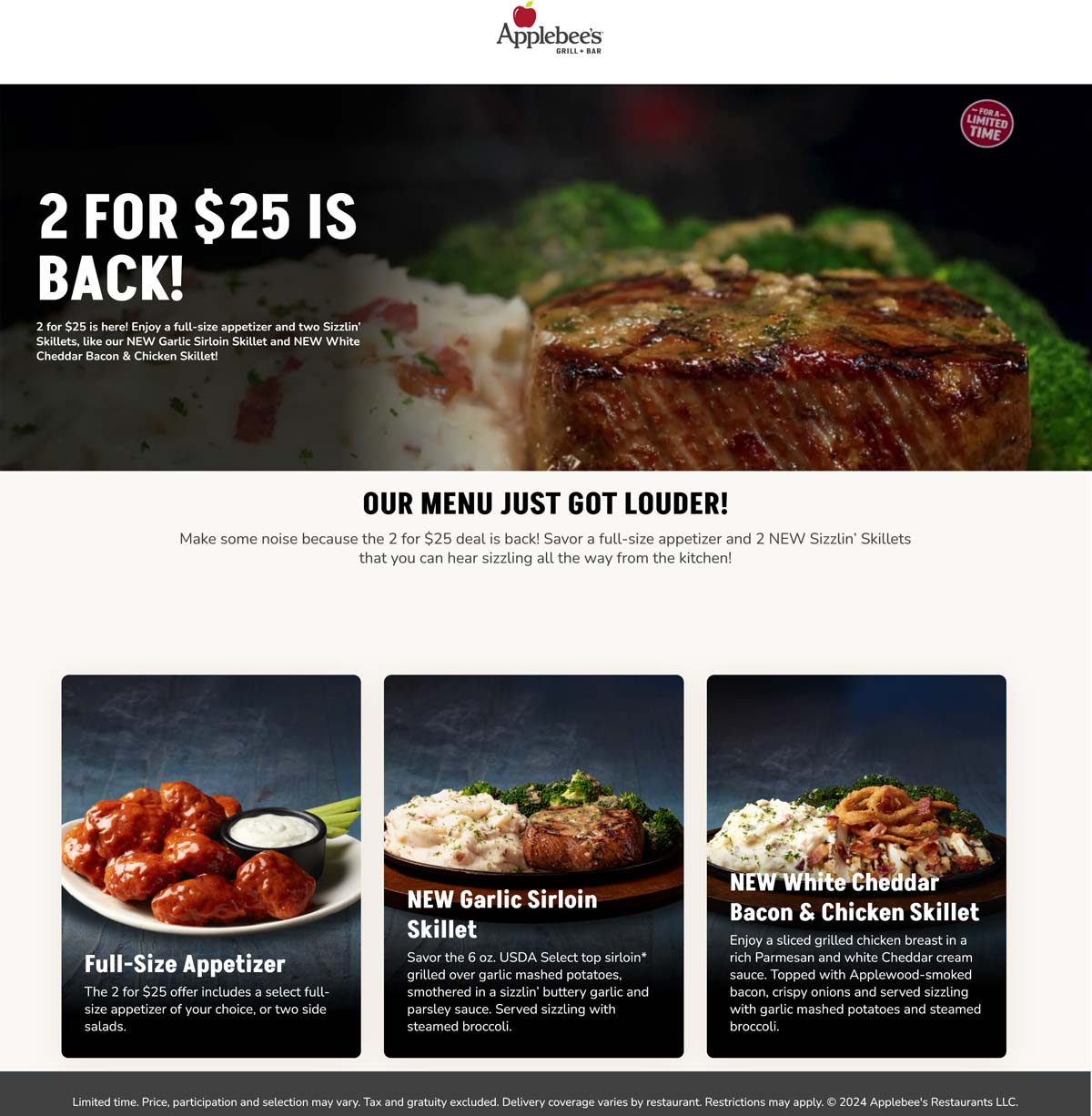**Applebee's Two for $2 Deal is Back!**

At the top of the ad, "Applebee's Grillin' Bar" stands out prominently. Below, a bold announcement catches the eye: "Two for Two Dollars is Back! Enjoy a full-size appetizer and two sizzling skillets, such as our new Chicken Sirloin Skillet and White Cheddar Bacon and Chicken Skillet." 

The ad features vibrant images of the dishes, starting with a detailed depiction of a color steak accompanied by steamed broccoli and creamy mashed potatoes. In the corner, a circular badge declares, "For a limited time," emphasizing the urgency of this special offer. Underneath, the slogan "Our menu just got louder" invites customers to make some noise about the deal. 

The "Two for $25" deal summary reads: "Savor a full-size appetizer and two new sizzling skillets that you can hear sizzling all the way from the kitchen." 

The bottom section of the ad includes three side-by-side images of the iconic dishes:
1. **Full-Size Appetizer:** A white plate piled with chicken bites drizzled in sauce, a small black ramekin filled with white dipping sauce, and celery sticks in the background.
2. **New Garlic Sirloin Skillet:** Features a 6-ounce USDA Select top sirloin, grilled and served over garlic mashed potatoes, drenched in a sizzling buttery garlic and parsley sauce, accompanied by steamed broccoli. It's presented on a black plate with a wooden charger.
3. **New White Cheddar Bacon and Chicken Skillet:** Showcases a sliced chicken breast in a rich parmesan and white cheddar cream sauce. It's topped with Applewood-smoked bacon and crispy onions, accompanied by garlic mashed potatoes and steamed broccoli. Presented on a black plate with a wooden charger.

At the very bottom, a small disclaimer reads: "Limited time offer. Price, participation, and selection may vary. Tax and gratuity excluded. Delivery coverage varies by restaurant. Restrictions may apply. ©2024 Applebee's Restaurants LLC."

Hurry in and take advantage of this mouth-watering deal before it’s gone!